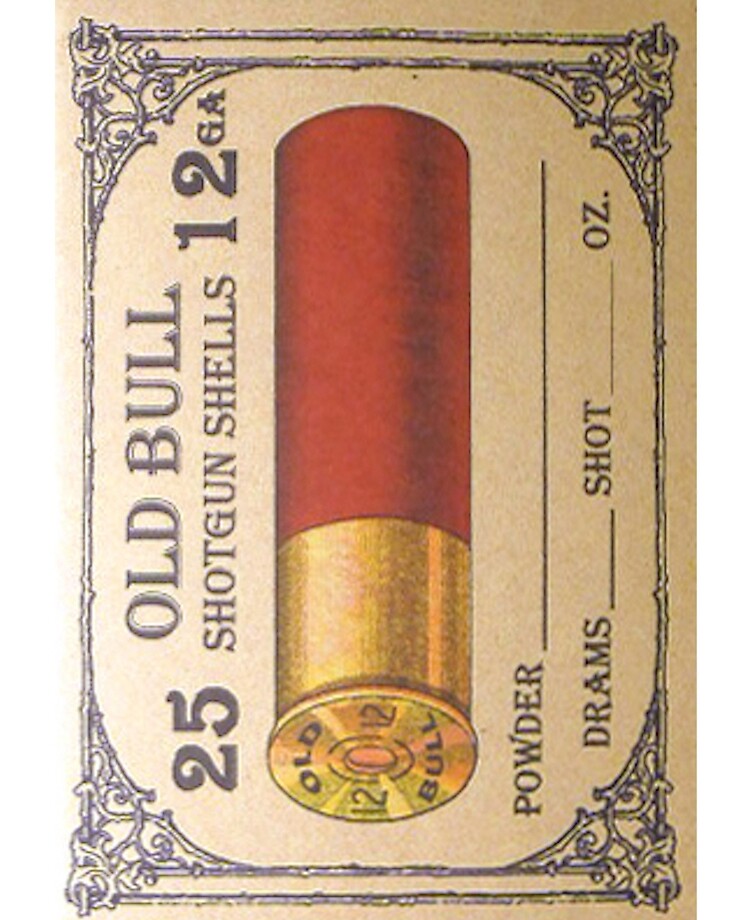The photograph depicts an aged, off-white box for Old Bull 12-gauge shotgun shells, likely turned vertically. The design features dark blue ornate bars and patterns accentuating the edges, giving it a vintage feel. Prominent black lettering announces "Old Bull Shotgun Shells" and "25 Shotgun Shells" in bold text. Centrally positioned is an illustration of a red shotgun shell with a gold base, the left lower part showing the label "Old Bull 12 GA". Beneath this drawing, there are blank lines with labels: "Powder", "Drams", "Shot", and "Ounce", intended to be filled out by the seller. The combination of the intricate border and detailed labels gives the box an authentic and textured appearance, standing out against its otherwise simple brown background.